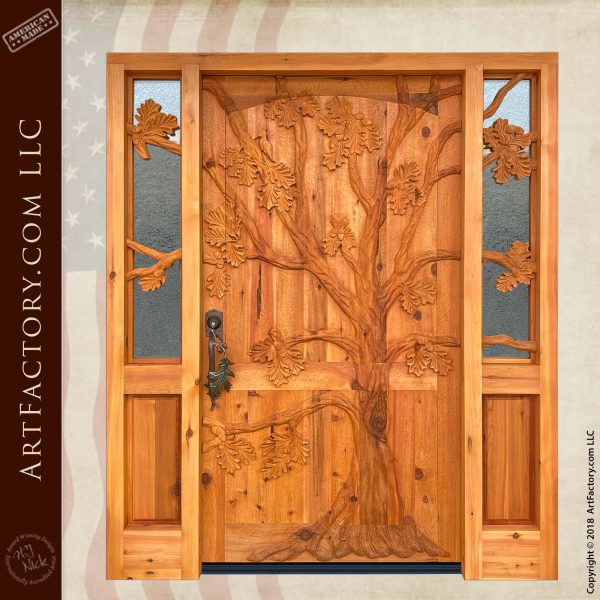This image appears to be an advertisement for a custom, hand-carved wooden door from ArtFactory.com LLC, copyrighted in 2018. The focal point of the image is a light brown, maple-colored door, intricately carved with a detailed tree design that spans the entire front of the door, with branches extending outward. On either side of the door are vertical wooden columns, topped with small glass panels that are partially obscured by wooden limbs extending in front of them. The door features a robust metal doorknob and handle, with a dangling artifact, possibly a leaf, suspended from a chain. The label "ArtFactory.com LLC" is displayed vertically along the left side of the image. Additionally, an understated silhouette of the American flag forms the background on the left, fading into a light gray on the right.